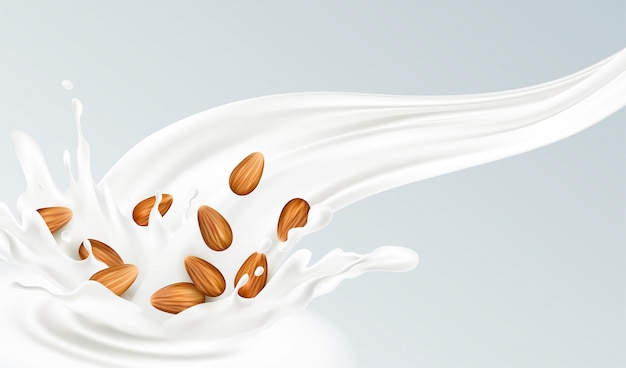This horizontal, digitally rendered image features a smooth, light grayish-blue background with a subtle green tint. Starting from the top right, a stream of white liquid, likely milk, flows leftward across the image, growing wider as it descends and splashes dynamically in the bottom left corner. The milk's splash sends droplets in all directions, creating a sense of movement and energy. In the midst of this splash, around ten light brown almonds, along with a few darker ones, are caught mid-air, enhancing the depiction of the liquid's impact. The absence of text in the image leaves the viewer to infer that this could be promoting almond milk, given the prominent inclusion of the almonds. One of the almonds is notably broken, adding to the realistic and captivating detail of the splash scene.